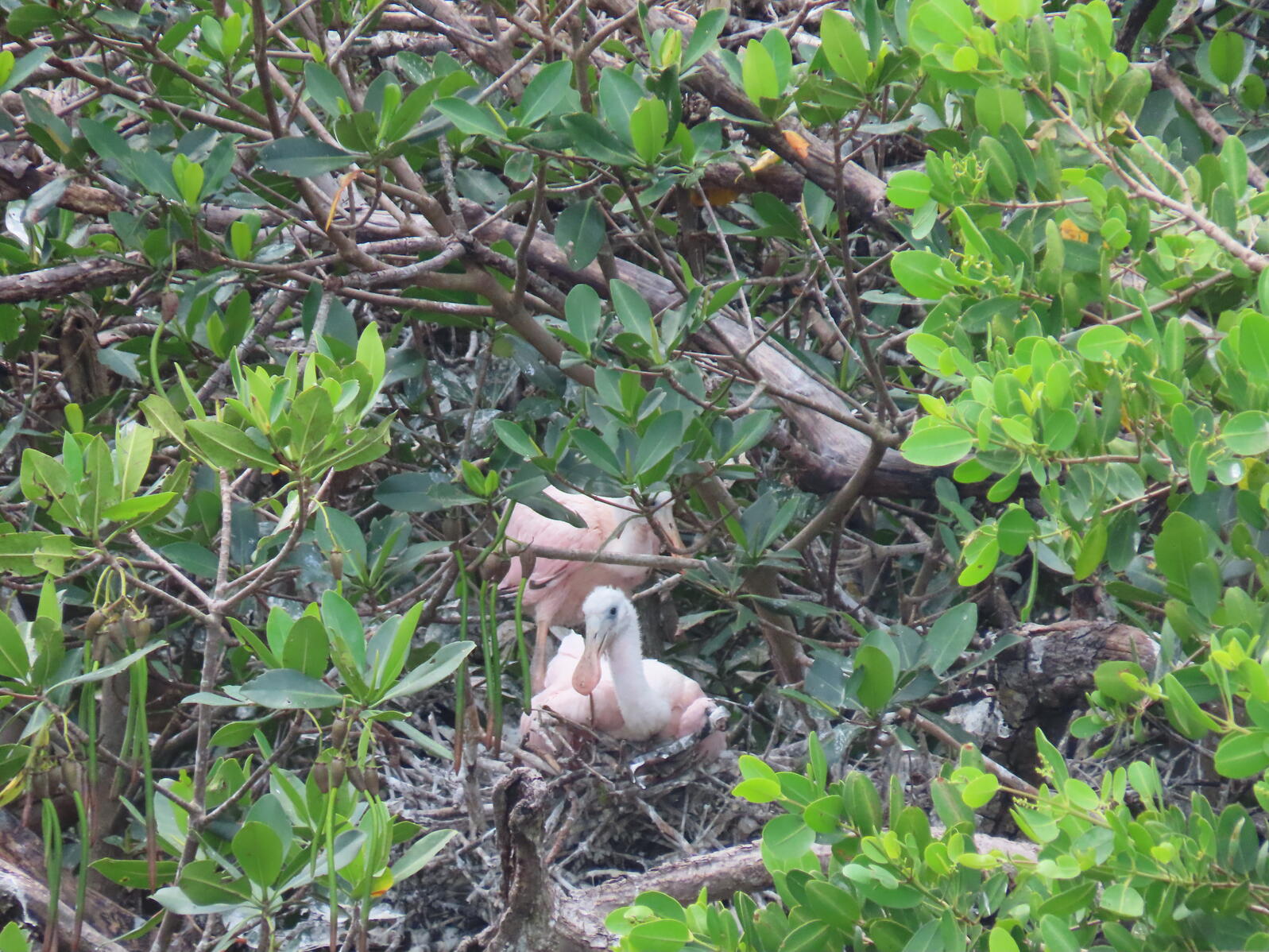In the photo, a densely wooded area filled with interwoven tree branches, stumps, and vibrant green leaves dominates the scene, particularly on the right side. The setting is tangled with brown branches and bushes dotted with bright green, oval-shaped leaves, some adorned with small yellow-orange flowers. At the center of this lush, natural tableau are two young birds resembling ducks, their bodies a light pink with pinkish, oval-shaped bills. The bird in the foreground, sitting, has a white neck and appears to be resting, while the bird in the background stands partly obscured by darker green leaves, seemingly hidden and blending into the dense foliage.